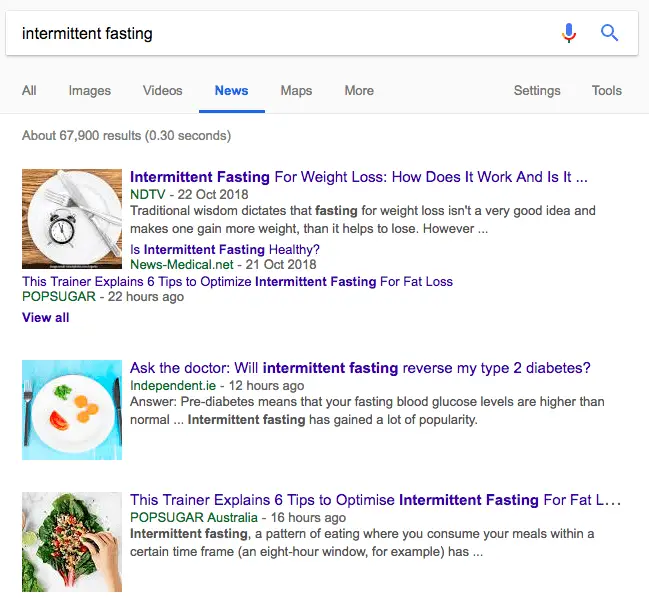On the search results page for "intermittent fasting," the top left corner features a search box where the term has been entered. Directly beneath the search box are various tabs for filtering results: "All," "Images," "Videos," "News," "Maps," and "More." The "News" tab is currently selected, highlighted in blue text with a blue underline, indicating the selection. Below this, the page indicates there are approximately 67,900 results.

The first result is titled "Intermittent Fasting for Weight Loss: How Does It Work?" but is truncated mid-sentence. The second result reads "Ask the Doctor: Will Intermittent Fasting Reverse My Type 2 Diabetes?" The third result is another incomplete title, "This Trainer Explains Six Tips to Optimize Intermittent Fasting for Fat L...".

Each search result is accompanied by a thumbnail image on the left. The first image shows a dinner plate with a spoon and a fork, along with an alarm clock. The second image features a white dinner plate with a fork and knife on either side, topped with eggs, tomatoes, and some greens. The third image displays a large leaf, possibly with a salad arranged in its center.